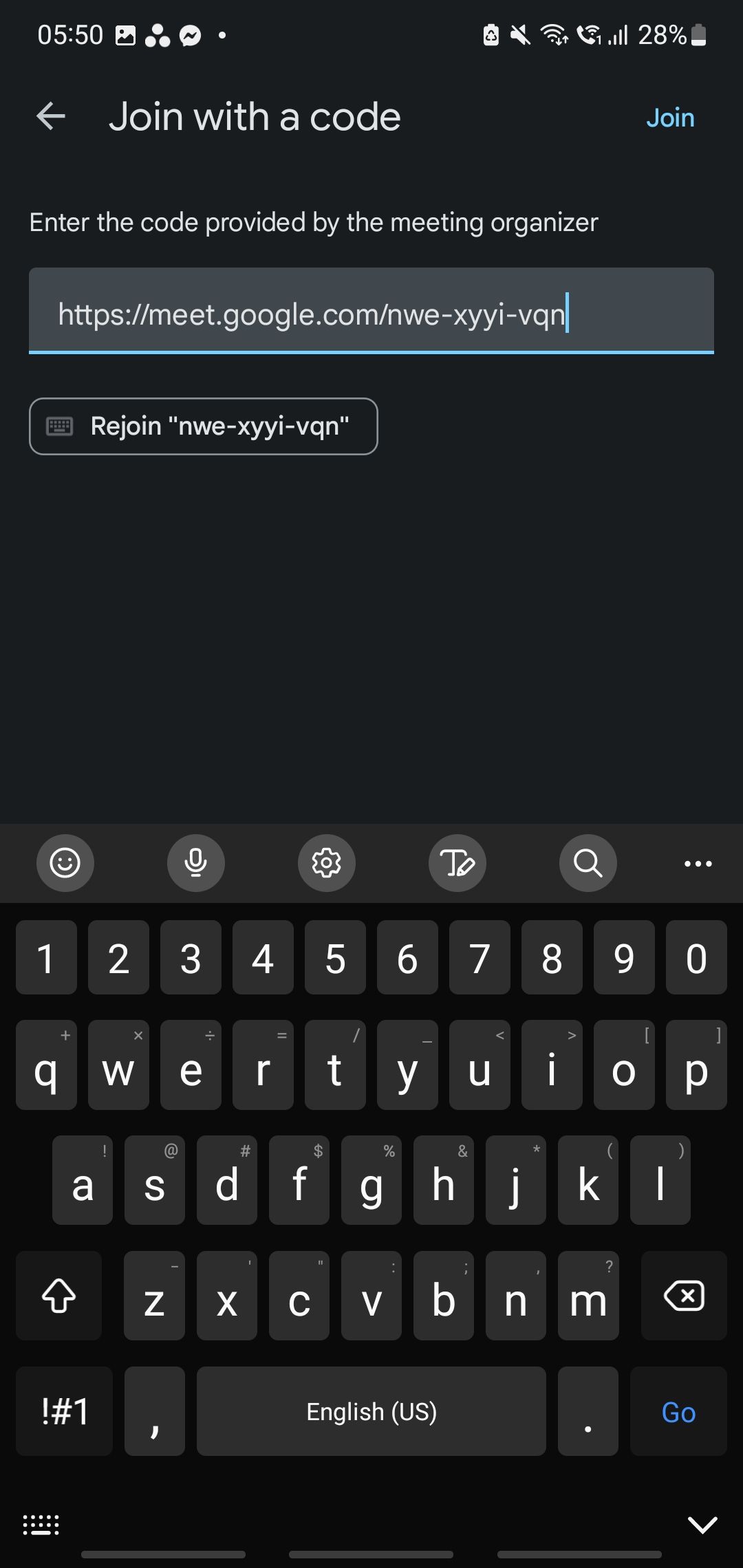This image, displayed on an iPhone, captures a screenshot of a Google Meet interface. In the upper left corner, the current time is shown as 5:50 PM, and the battery life is at 28%, accompanied by other standard status icons. 

At the top of the screen, a black bar prompts the user to "Enter the code provided by the meeting organizer." Beneath this, the URL "meet.google.com" is highlighted with a blue underline and a vertical blue line at the end, matching the shade of the "join" button on the right side of the screen. 

There's a large text input field prompting the user to "Join with a code," with a left-pointing arrow to its left, and a prominent blue "Join" button on the right. Below this, there is a "Rejoin" button for easy reconnection to previous meetings. 

At the bottom of the screen, the iPhone's black and white keyboard is visible, complete with all standard text input keys. The interactive interface is highlighted by a "Go" tab in blue and an arrow pointing downward, indicating further options. On the left side of the keyboard, there is a dot and a screen icon, providing additional functionalities for the user.